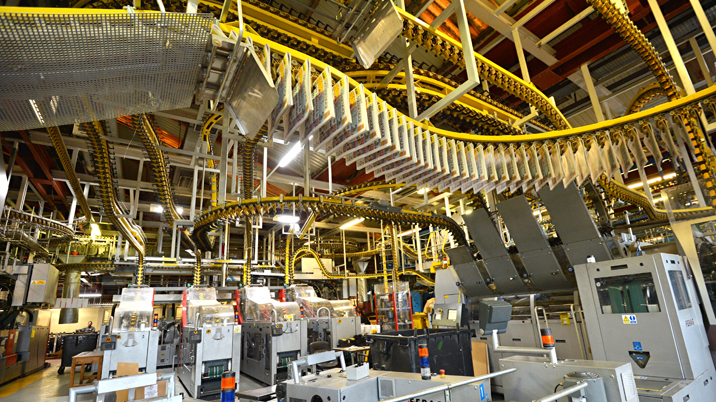The photograph captures the bustling interior of an automated industrial factory. The scene is dominated by a yellow metallic conveyor belt system that intricately winds around the ceiling, reminiscent of a roller coaster track. Suspended from the conveyor are large, filter-like objects, approximately two feet by three feet, each securely clipped as they move through various stages of processing. The ground level is populated with a variety of unfamiliar, boxy industrial machinery, many with glass-fronted, white metal cabinets, likely designed to allow observation of internal operations. The factory is crisscrossed with a network of white and red beams, adding to the complex, almost circus-like ambiance. Despite the lack of visible workers, the facility appears to be fully operational, efficiently transporting and processing materials through its extensive automated systems.